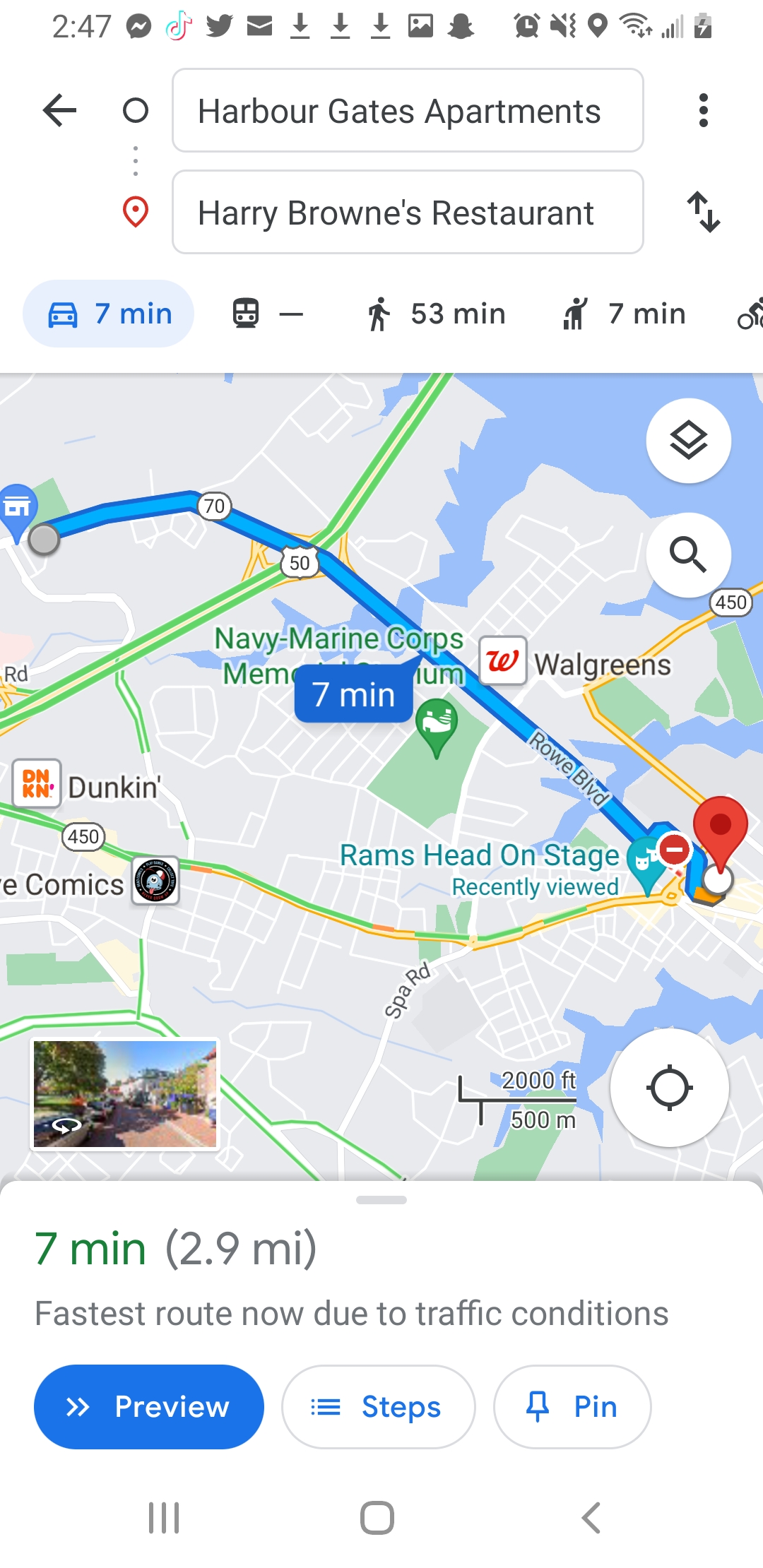This detailed screenshot, taken from a smartphone, shows Google Maps displaying a route from Harbor Gate Apartments to Harry Brown's Restaurant. The image features a light gray map with roads depicted in white, a body of water in light blue in the upper right corner, and highlighted roads in green and yellow. The route is marked in bright blue, with a speech bubble indicating a travel time of seven minutes. At the top of the screen, a menu lists the starting point, Harbor Gate Apartments, and the destination, Harry Brown's Restaurant. Below the map, additional information reads "7 minutes (2.9 mi)" in green, followed by "fastest route now due to traffic conditions" in gray. Three buttons—Preview (shaded in blue), Steps, and Pin with a pin symbol—are situated beneath this text. A thumbnail image of the destination and a white turnaround symbol can also be seen on the bottom left-hand corner of the screen. The map includes standard Google Maps outlines, providing a visual guide of the journey.